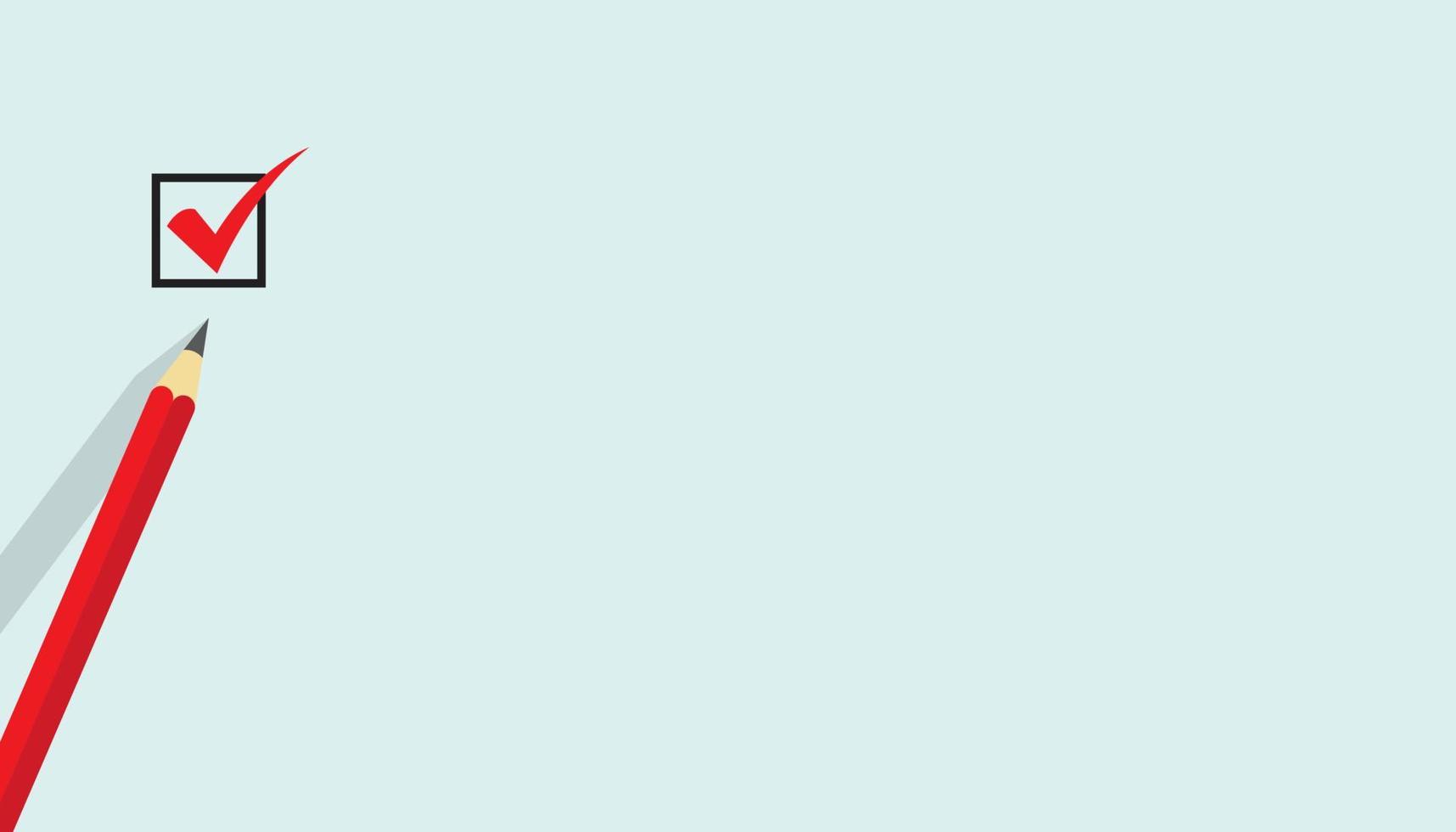The image features a computer-generated graphic set against a light robin's egg blue background that could serve as wallpaper or a website banner. On the left side, a detailed, cartoon-like red pencil with a sharp, dark slate gray tip is depicted, leaning diagonally with a shadow cast underneath. Slightly above the pencil, in the upper left corner, is a black square containing a prominent red checkmark. The pencil does not appear to have made this red checkmark, as the tip color is a dark gray, creating contrast within the image.